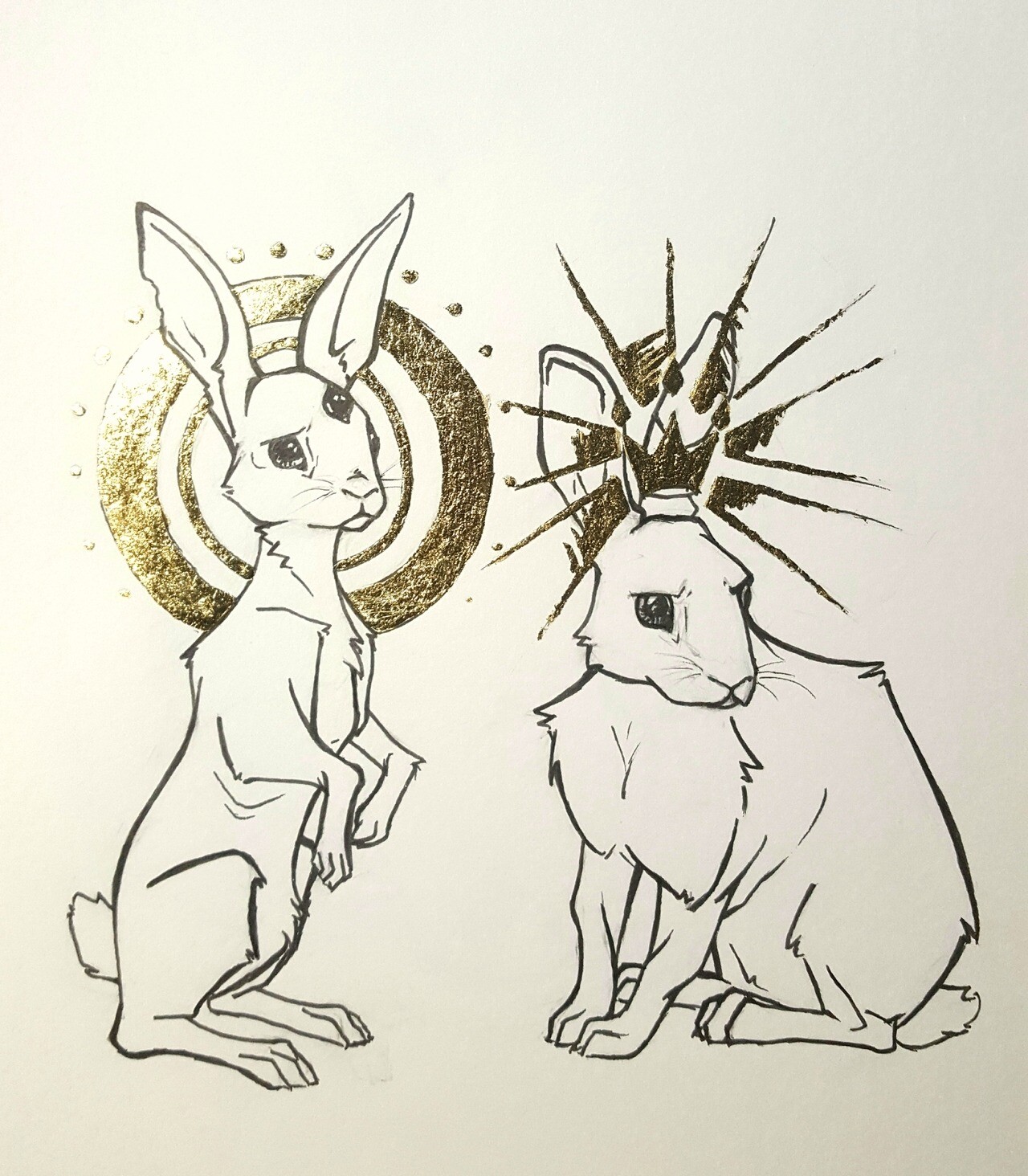This rectangular black and white sketch features two long-eared, furry rabbits with triangular faces and big eyes, set against an off-white background. The rabbit on the left stands upright on its hind legs, with its front paws raised and its ears up in the air. Uniquely, this rabbit has an extra eye on its forehead, encircled by a gold halo consisting of two concentric circles with golden dots around the outer, thicker circle. The rabbit on the right sits with all four paws on the ground, its body turned to the left while it looks to the right. This rabbit wears a glistening gold, three-pointed crown adorned with starburst-like golden rays emanating from it. Both rabbits are rendered in bold black lines, with gold highlights accentuating their features.